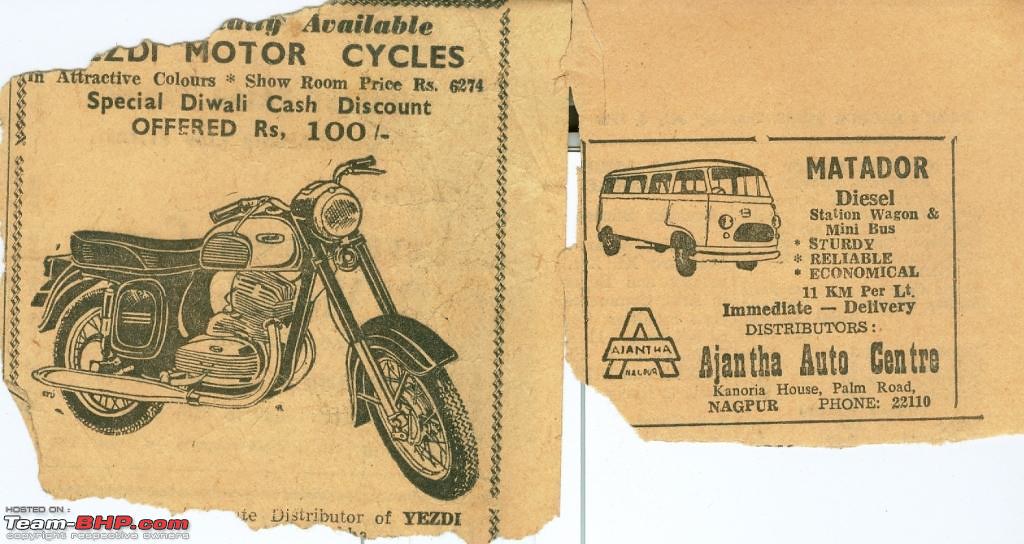This image features a torn, yellowed newspaper with vintage advertisements. On the left panel, there is a black-and-white illustration of a motorcycle bordered by a frame. The visible text reads: "Available motorcycles in attractive colors, showroom price RS6274, special Diwali cash discount offered RS100." The brand "Zeddy" is mentioned, and it notes the distributor "ESD." On the right panel, there is an advertisement for a VW van, specifically a 15-seater minibus. It states: "Matador diesel station wagon minibus, sturdy, reliable, economical, 11 kilometers per liter, immediate delivery." It lists the distributor as "Ajanta Auto Center, Penoria House, Palm Road, Nagpur," with the contact phone number "22110." The overall presentation of the newspaper indicates it has aged with time, giving a peek into the past with its vintage ads.